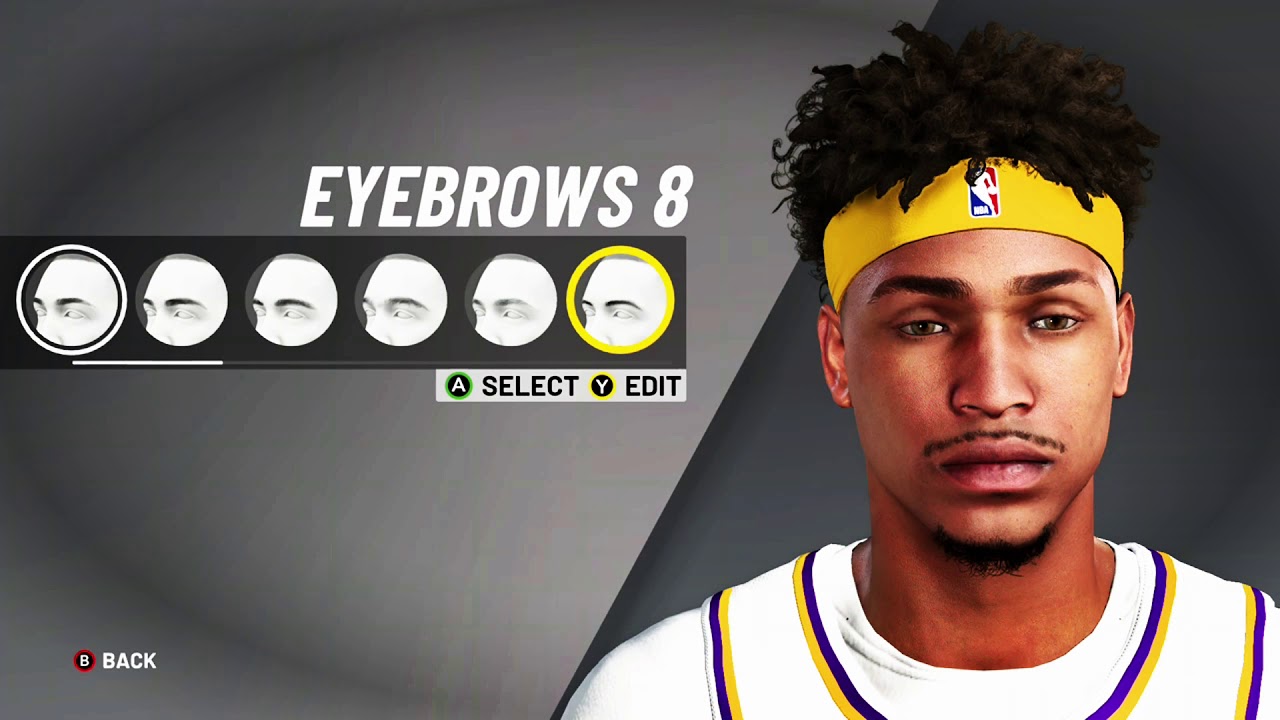This rectangular image features a character customization interface with a visually layered background transitioning from light gray to medium gray to dark gray. 

On the left side, the word "Eyebrows" is prominently displayed in bold white text, followed by "8" beneath it, also in white. Below this text, there's a rectangular box showcasing a selection of eight different eyebrow styles. The eighth option, positioned on the far right, is highlighted with a yellow circle.

Underneath this selection box, a light gray panel provides control instructions: "A to select" or "Y to edit." The "A" button is indicated by a green circle, while the "Y" button is highlighted with a yellow circle. At the bottom left corner, a black circle with a red outline contains a white "B" labeled "Back."

On the right side of the image stands the avatar: a black man wearing a yellow headband that wraps around his forehead just above his ears, keeping some of his hair in place. He gazes straight ahead with a neutral expression, sporting a thin mustache and a modest goatee. His attire consists of a white undershirt, over which he wears a white jersey trimmed with purple and gold accents.

The image captures the moment of customizing the avatar's appearance, specifically selecting eyebrow styles.